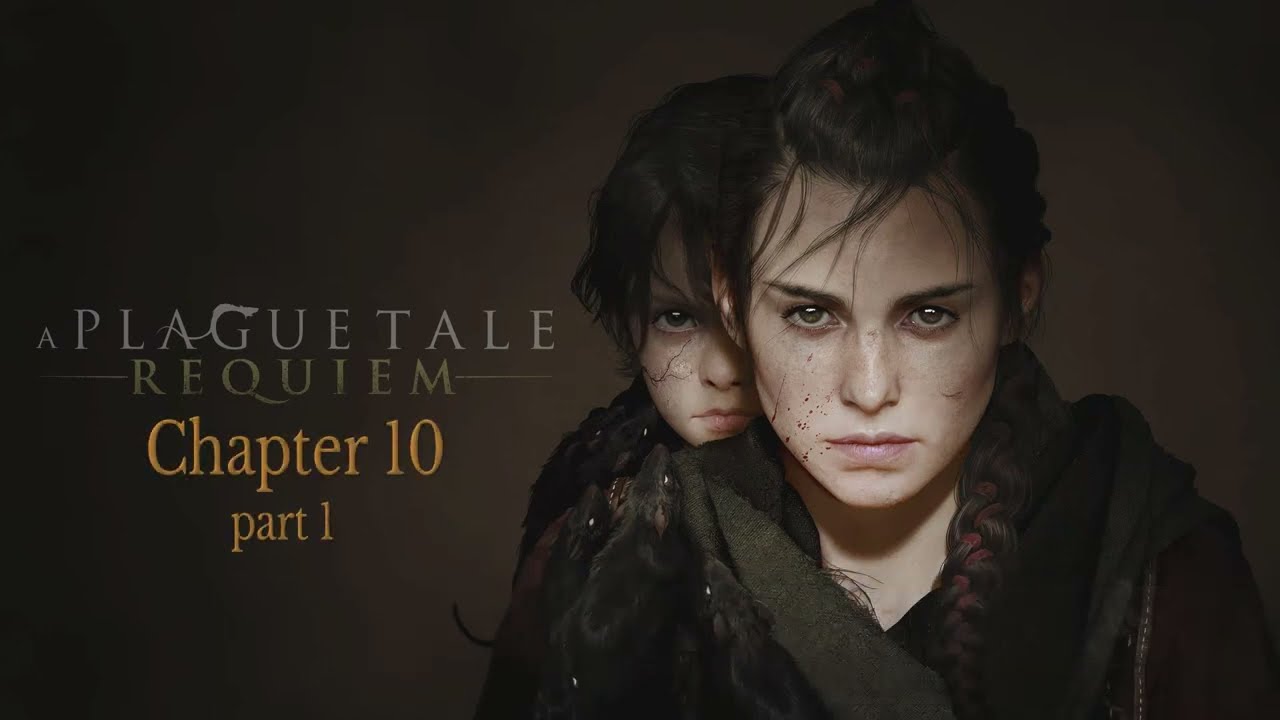The image features a detailed and intense scene that appears to be a promotional screenshot for a chapter of a story, possibly a fiction novel, movie, or TV show. Dominating the right side of the image are two figures: an adolescent girl and a younger child. The girl, with a pale complexion, has brown hair tied in a braid over her left shoulder, which has red tinges in it. She wears dark brown clothing and has a serious, possibly frightened expression. The child is positioned behind her, looking over her right shoulder with a similar dour expression. The color palette includes brown, green, red, gray, yellow, pink, and black, lending a somber tone to the image. The background is predominantly a solid brown. On the left side, there is text that reads: "A Plague Tale Requiem, Chapter 10, Part 1," with 'Chapter 10, Part 1' highlighted in yellow. This vividly descriptive scene seems to be an advertisement or promotional material for "A Plague Tale Requiem."